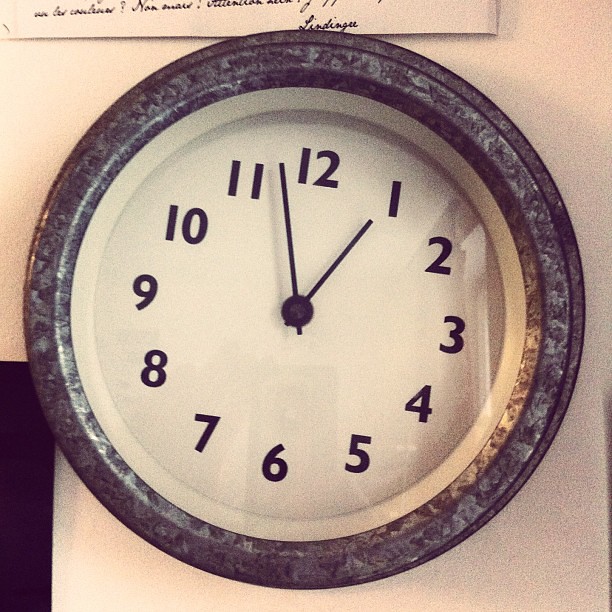A detailed photograph showcases a circular wall clock prominently positioned slightly off-center and tilted to the right. The clock features a white face with black numerals and black clock hands indicating the time as 12:58. There is a noticeable reflection on the clock's glass covering. Above the clock, an artistic painting adorns the wall, featuring black cursive inscriptions in a different language and a signature at the bottom. The painting hangs on a clean, white wall, contributing to the minimalist aesthetic of the scene. In the lower left corner of the photo, a black bar juts out, suggesting another wall feature or hanging. The overall setting emphasizes simplicity and subtle artistic elements.